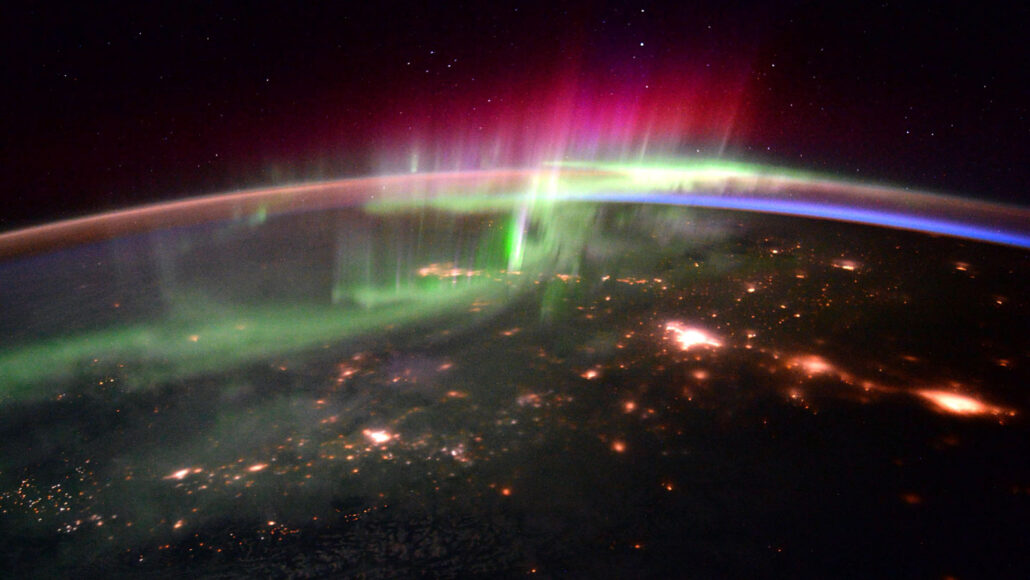This stunning image, captured from space, showcases a nighttime view of Earth illuminated by city lights glowing in shades of orange and red, giving the appearance of fiery magma or hot embers. Above this dazzling earthly display, an ethereal aurora borealis spreads across the horizon with misty hues of green, pink, and red, accompanied by sharp blue lines and white accents. The scene is framed by the infinite blackness of space, dotted with small, distant stars, creating a majestic contrast between the vibrant activity on Earth and the serene stillness of the cosmos.